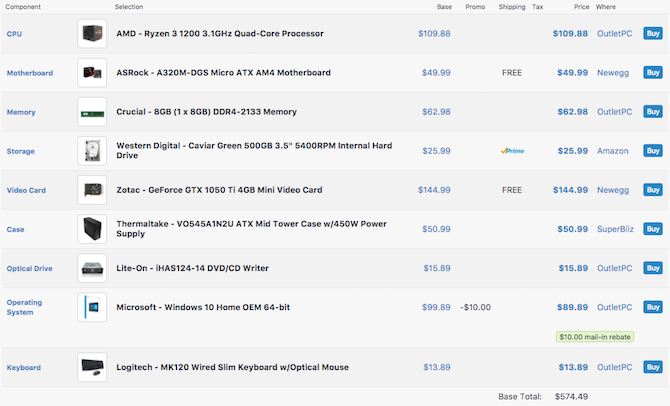The image features an all-white background with a blue hue. In the top left corner, small letters read "Component." Directly underneath, various system components are listed in blue text: CPU, motherboard, memory, storage, video card, case, optical drive, operating system, and keyboard. Each component is separated by thin lines, forming individual rectangles. 

To the right of this list, a section labeled "Selection" displays the chosen product's name. Adjacent to the product name, there is a white square containing a picture of the product. To the right of the image, the word "Base" is prominently displayed in black text. Below it, the price is listed in blue.

One of the rows includes a notation reading "Promo," and beneath it, a line indicates a $10 discount in black text. Near the top, the word "Shipping" is listed with the second row indicating "Free." The fourth row displays "Prime," while the fifth row states "Free." The section labeled "Tax" remains empty, and the subsequent "Price" section shows the amount in blue.

On the right side of the image, vertical blue tabs with white letters read "Buy." The eighth tab down, second from the bottom row, features a gray tag with "Mail-in Rebate" in black text and a black border. The final price, $574.49, is displayed in black text at the bottom, next to the label "Base Total."